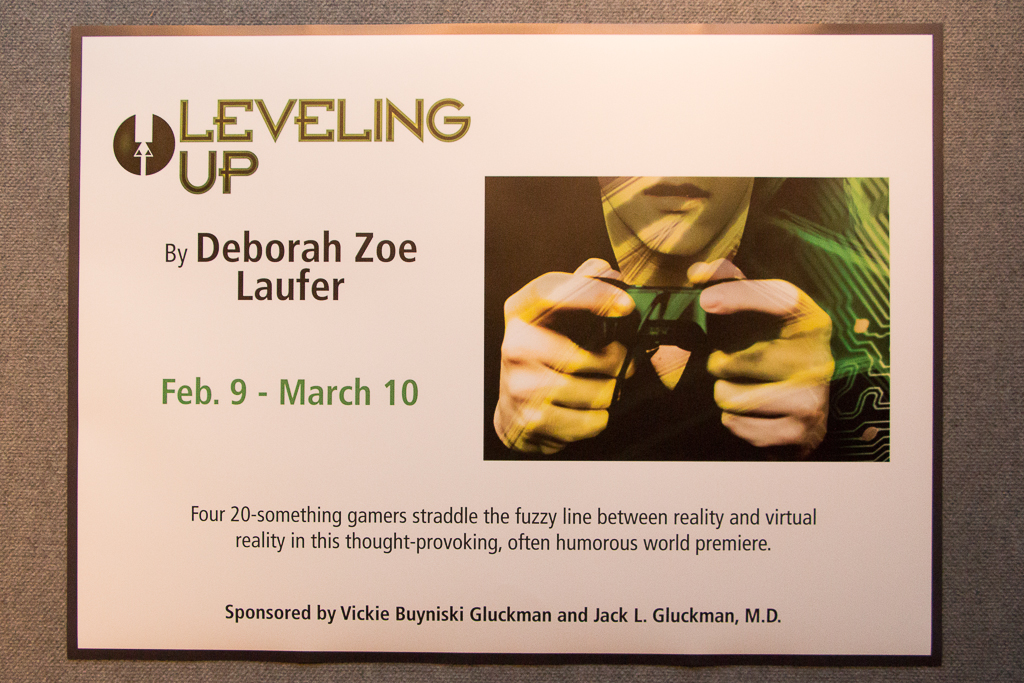The image portrays a detailed poster set against a purplish-brown burlap-like cloth background. The poster has a border matching the cloth’s color, with "Leveling Up" prominently displayed at the top. Authored by Deborah Zoe Laufer, the event runs from February 9th to March 10th, with these dates marked in green font. 

On the right side of the poster, there is an image of a person captured from their lips down to their chest, holding a black video game controller with a wire. This section is juxtaposed with the description of the play, which reads: "Four 20-something gamers straddle the fuzzy lines between reality and virtual reality in this thought-provoking, often humorous world premiere." 

The sponsorship is credited to Vicki Bunewski Gluckman and Jack L. Gluckman, MD. The entire composition conveys a nuanced blend of visual and textual elements, intricately interwoven to emphasize the play’s themes and contributors.